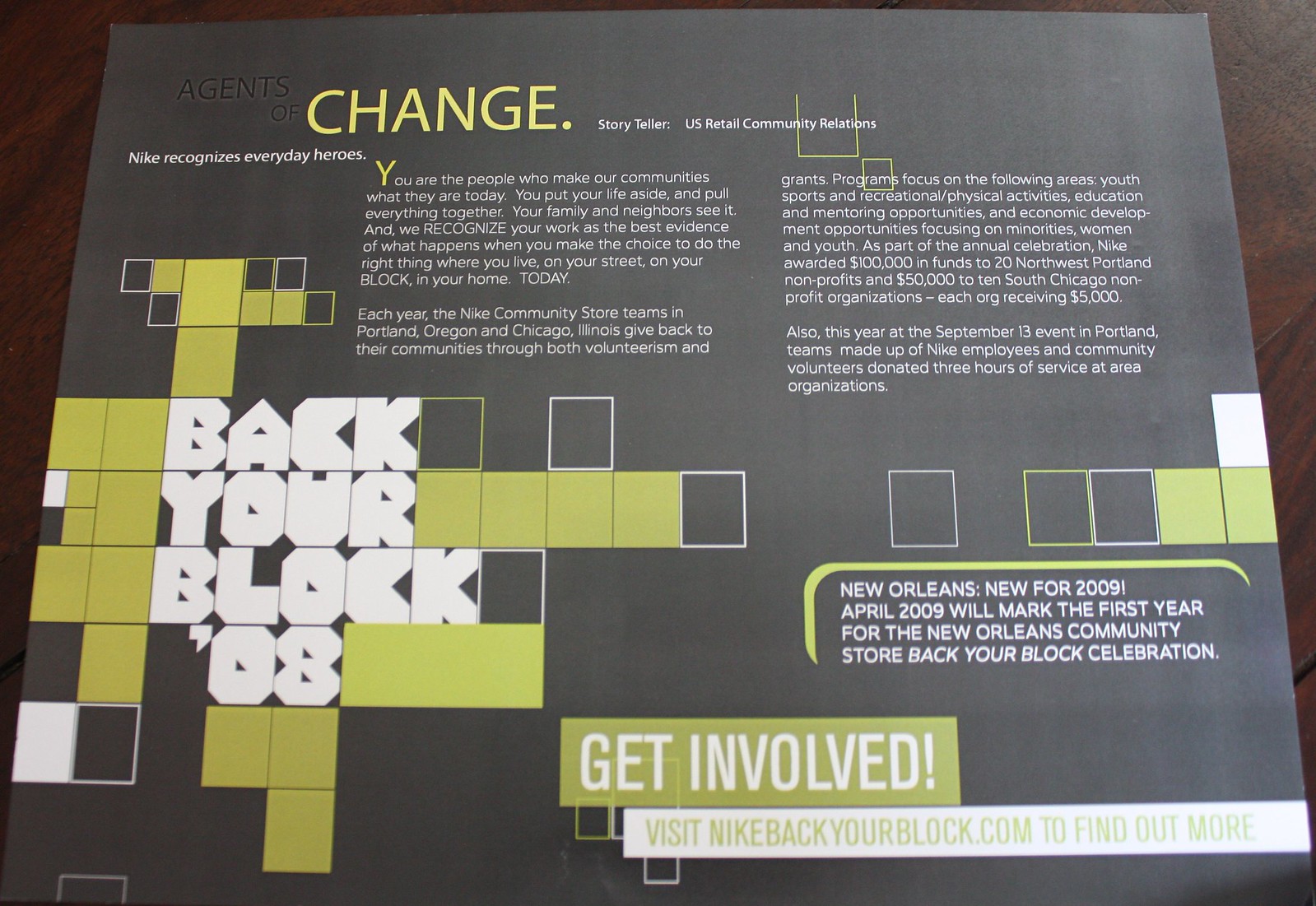The image is an advertisement poster from Nike with a dark gray background, featuring a mix of white and lime green text. At the top left, it prominently states "Agents of Change" with "Change" highlighted in lime green. Adjacent to this, it reads "Storyteller, U.S. Retail Community Relations." The poster recognizes everyday heroes, emphasizing the role of community members in shaping their neighborhoods. It includes a detailed message about Nike's commitment to community service, noting that Nike Community Store teams in Portland, Oregon, and Chicago, Illinois, annually engage in volunteer work and provide grants. Specifically, $100,000 and $50,000 were awarded to non-profits in these cities, respectively, with each benefitting organization receiving $5,000. The content highlights various focus areas such as youth sports, physical activities, education, mentoring, and economic development, particularly targeting minorities, women, and youth. The poster also announces the initiation of the New Orleans Community Store "Back Your Block" event starting in April 2009. Decorative elements on the left side of the poster use interconnected blocks spelling out "Back Your Block 08" and draw the eye towards the information, culminating in a call-to-action at the bottom right, urging viewers to visit nikebackyourblock.com for more information. The layout is modern and visually appealing, blending text and graphic elements effectively to convey Nike's CSR initiatives.